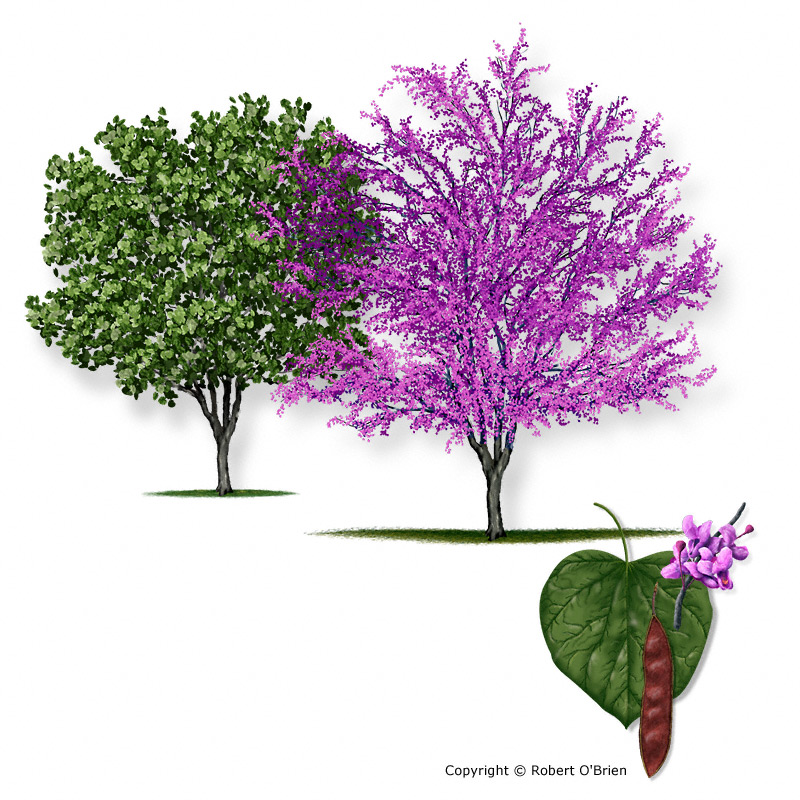This image is a detailed artistic drawing of two trees set against a bright white background. The tree on the left is fully matured with lush, dark green leaves emerging from a narrow brown trunk, suggesting it is in full bloom during summer. In contrast, the tree on the right features sparse, pinkish-purple leaves, indicating it is in the budding phase of spring. Both trees are of similar size and appear to have been hand-drawn or digitally illustrated rather than photographed.

At the lower right corner of the image, there is a depiction of a green leaf with a purple flower at its upper corner. Overlapping this leaf is a brown, pea pod-shaped container that seems to contain seeds or buds. The bottom of the image displays the text "© Robert O'Brien" in black lettering, indicating the copyright information for the artwork.

Overall, the image is bright and clear, showcasing vivid colors and fine details that contribute to its diagram-like quality.